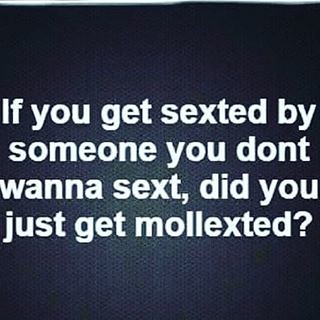In this square-shaped image, there is no physical object, only text presented on a predominantly black or dark blue background. The design features four lines of bold, white, sans-serif lettering centered in the middle of the image, with the text slightly extending to the edges on both sides. The message humorously reads, "If you get sexted by someone you don't want to sext, did you just get malexted?" This typographic composition combines elements of graphic design with a satirical meme style, likely intended for sharing on social media. The image maintains a minimalist aesthetic, focusing solely on the text without any additional visuals.